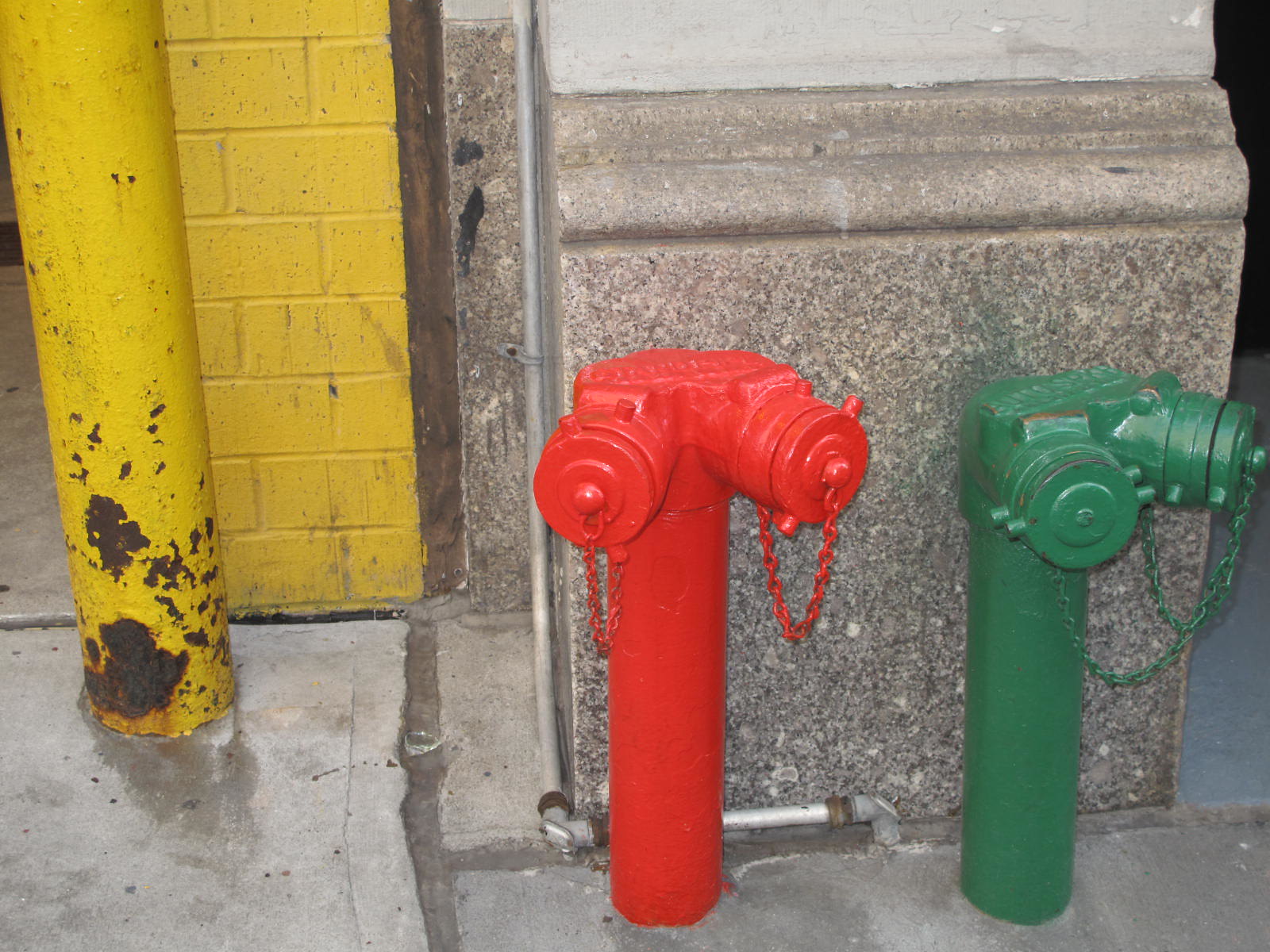The color photograph captures a grimy urban scene featuring vivid hues of yellow, red, and green. The setting appears to be part of a subway system or city infrastructure, showcasing a tight close-up view of two fire hose spigots mounted on a sidewalk. These spigots, not traditional fire hydrants, consist of vertical posts with Y-bracket splits, allowing for two capped outlets each. The left spigot is painted bright red, while the right one is painted forest green. Both have caps attached with chains. To the left of these spigots, a yellow-painted brick wall with a thick, rust-exposed yellow metal bollard stands out. The area above the ground level features a gritty cement or concrete facade, partially covered by a granite section extending three to four feet upward. Behind the fire hose spigots, a thin metal pipe runs parallel to the wall, adding to the industrial and worn-out atmosphere of the scene. The overall composition highlights the contrasting textures and colors, from the chipped paint to the rough concrete, creating a detailed and vividly gritty urban snapshot.